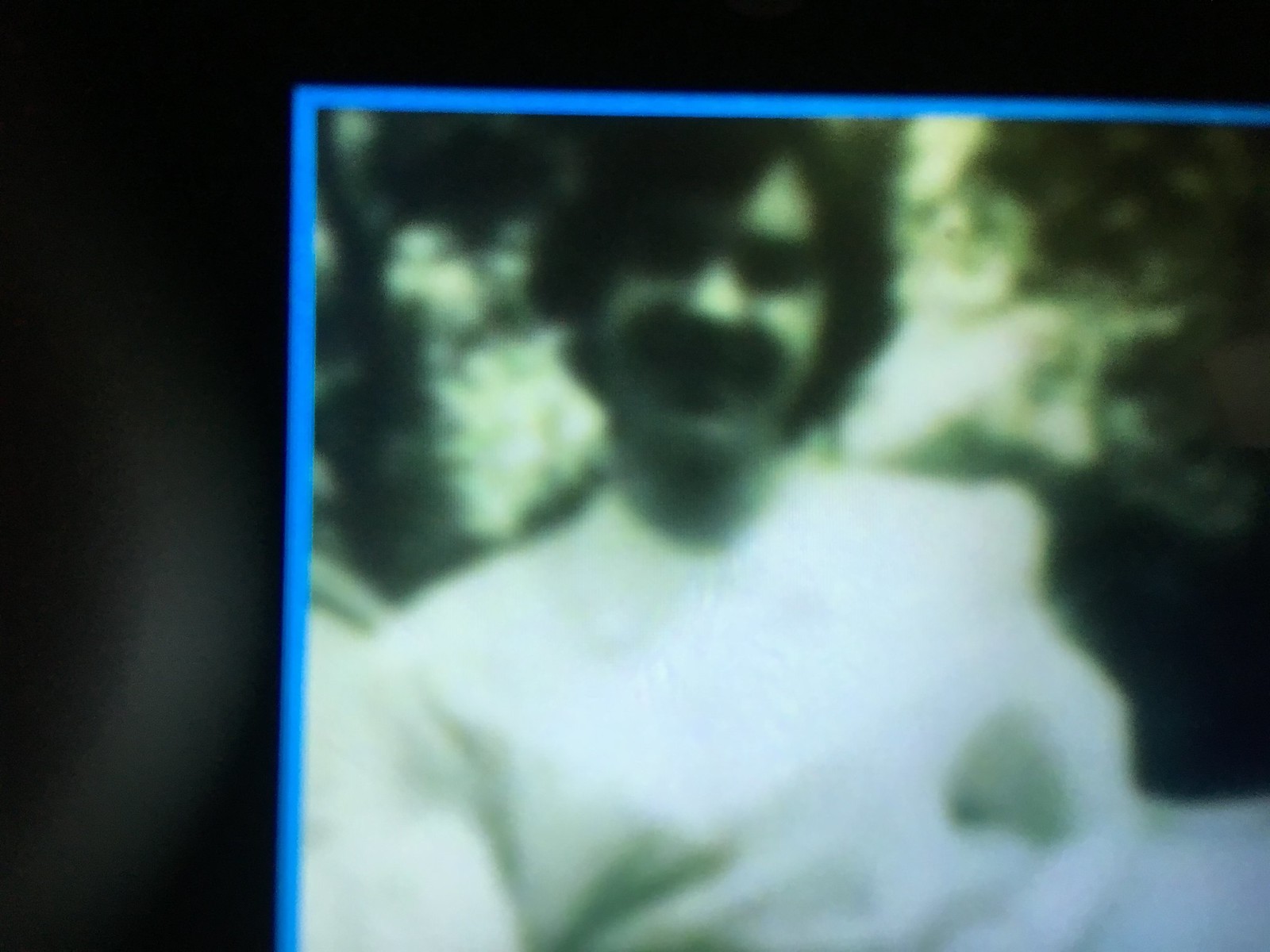This is a blurry, monochromatic photograph with a distinct greenish tint, likely indicating it was taken from a digital device like a computer screen. The image features a smiling man with longish dark hair that covers his ears and a mustache. He wears a white, long-sleeve, button-up shirt. Shadows obscure his eyes. The background of the photo shows some trees and greenery. A bright blue line outlines the upper left corner of the photo, while the rest of the edge is obscured, suggesting only a portion of the original photograph is visible. The photo itself is set against a black background, adding to the observed dark tones.